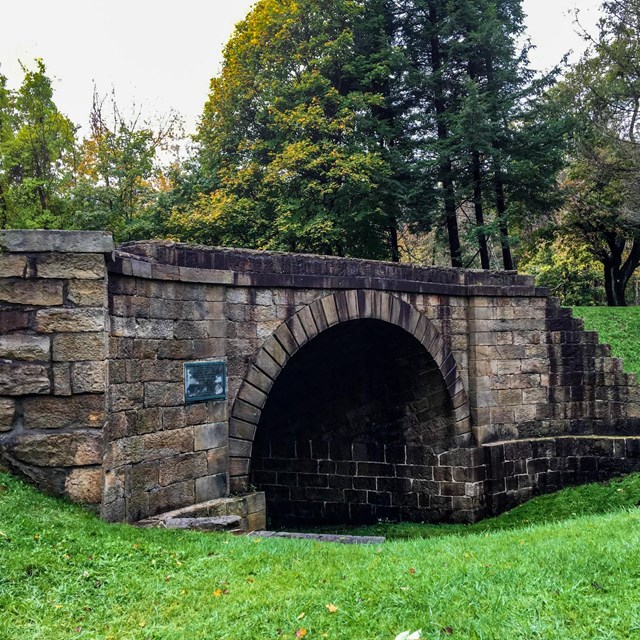This outdoor photograph captures an old stone bridge with a prominent archway leading into a dark, tunnel-like underpass. The bridge, made of weathered sandstone or brown brick, shows signs of age with missing bricks and natural stains. An unreadable plaque of dark green or bronze is visible near the top left of the tunnel mouth. The setting is a lush, well-maintained lawn, surrounded by a mix of tall green trees and shorter foliage, suggesting a late summer or early fall season. The sky above is a mix of grayish-blue and white, enhancing the serene ambiance of this seemingly abandoned, yet tranquil, park-like area. Steps on the right side of the bridge descend into the grassy foreground, hinting at a pathway for pedestrians.